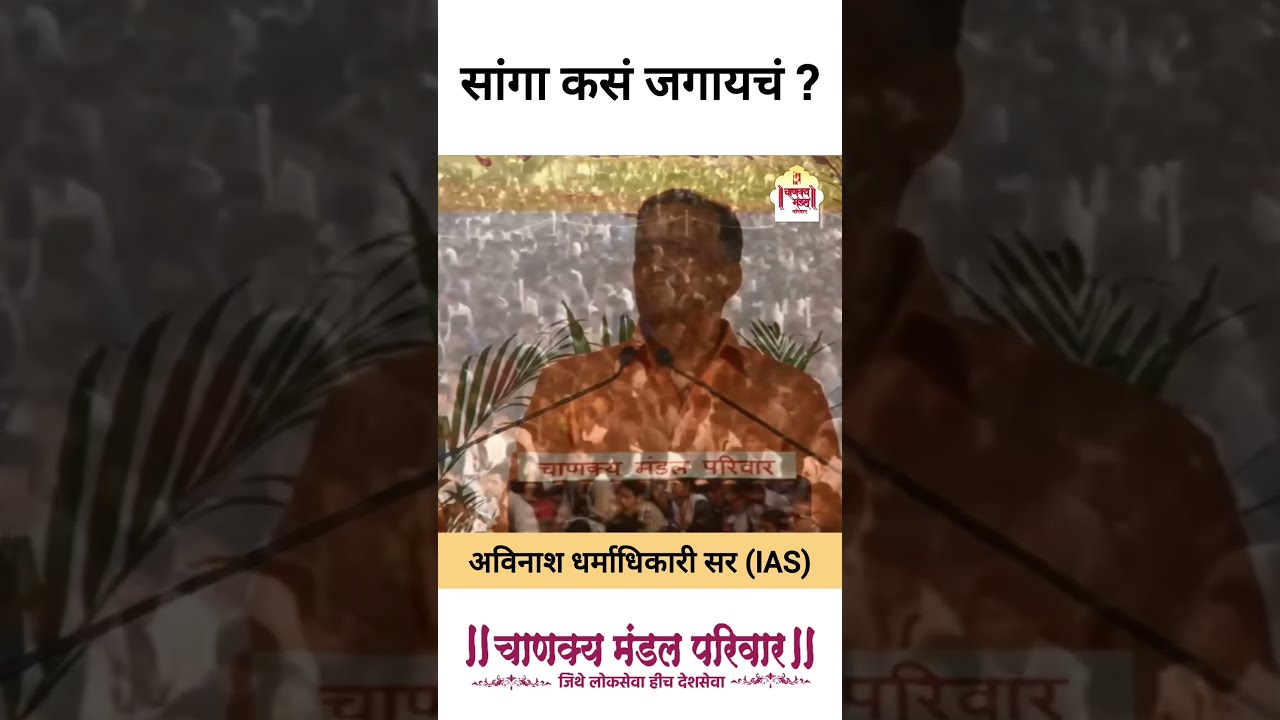The image is a rectangular poster, approximately six inches wide and four inches high, divided into three vertical sections. Dominating the center section is a slightly pixelated image of a man with dark skin and very short black hair, wearing an orange button-up collared shirt. He stands amidst a background featuring a watery texture effect and darker greenish-brown hues, with slender plant leaves encircling him.

At the top of the center section, there is Arabic text, identifiable by its curly lines, straight lines, and dots. Beneath the man's image, there is a gold strip with more Arabic text, followed by a white rectangle also containing Arabic script in maroon and red colors. The letters "IAS" appear within the gold strip. To the left and right sections of the poster are enlarged and darkened images of the man, showing close-ups of his shoulders and the crowd of people behind him. The harmonious overlay of these elements suggests a message of unity and engagement.